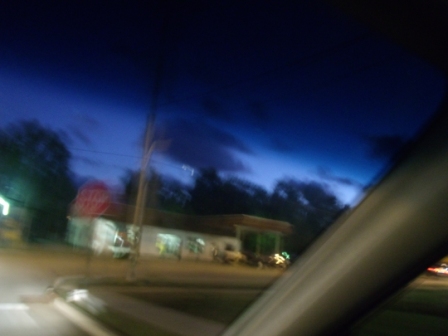This nighttime outdoor image, captured through the windshield of a vehicle with a gray or tan interior frame visible on the right, shows a blurred but evocative scene. The upper third of the windshield appears tinted, casting a darker shade over the sky, which transitions to a lighter blue hue near the horizon. This lighter portion illuminates the outline of a cloud. Directly across the street is a business with a distinct red roof and white walls, resembling a diner or convenience store. To its right, a carport-style structure is present with two vehicles parked underneath. Dense, dark trees form a silhouette behind the building. A stop sign is visible near the business, and the car's headlight emits a soft white light, faintly illuminating the road ahead.